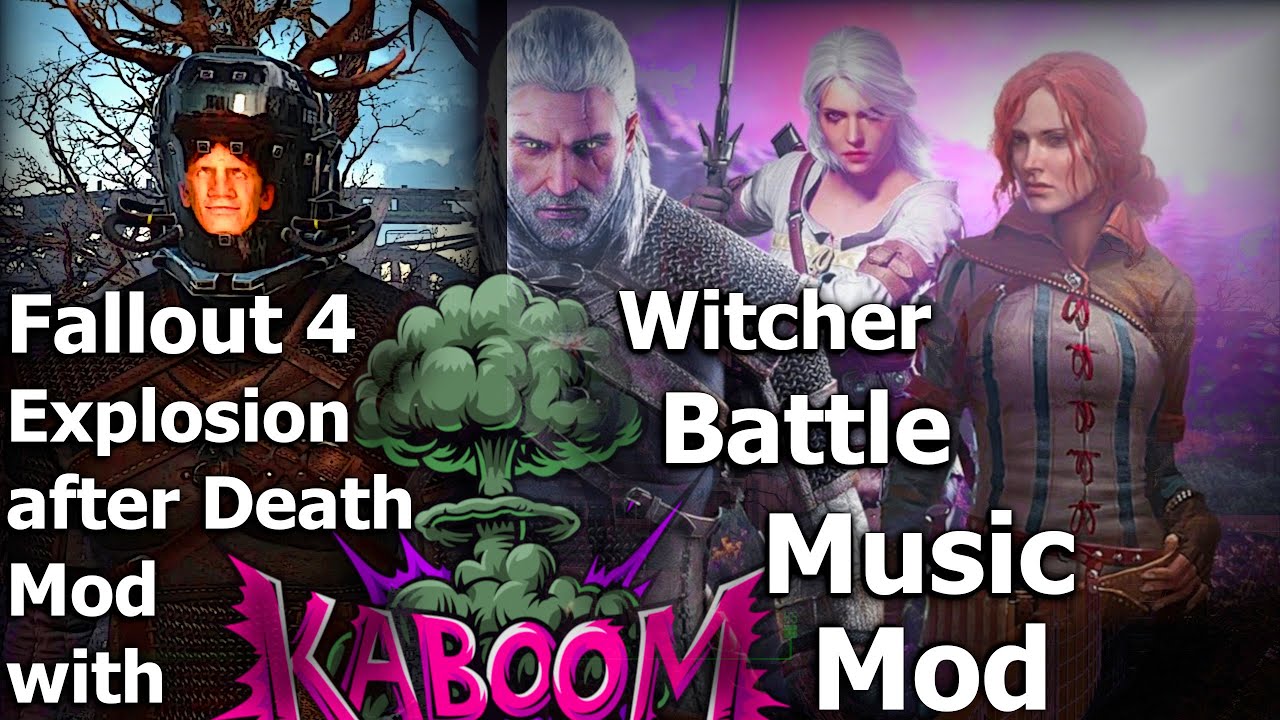This image, likely from a video game advertisement, is split into two distinct sections featuring prominent characters and text. On the left, a character clad in an exoskeleton with dark brown and metal plating stands before a bare tree with background structures visible. This figure is associated with the "Fallout 4 Explosion After Death Mod," displayed in white letters across his chest. Dominating the center, a vivid green mushroom cloud rises with the word "Kaboom" in bold pink, surrounded by purple rays that highlight the explosion’s intensity.

To the right, the focus shifts to characters from "The Witcher Battle Music Mod." Central to this section is a silver-haired man with piercing eyes, a beard, and a distinctive scar running from his forehead to his cheekbone, dressed in substantial armor. To his left is a young woman with stark white hair, dressed in a flowing white outfit, raising a silver sword in her right hand. Beside her stands a redheaded woman in a multicolored outfit featuring vertical greenish-blue stripes, red strings tying the shirt's front, and a diagonally draped shawl around her shoulders. The juxtaposition of these characters, enhanced by the detailed costumes and dynamic background elements, underscores the dramatic and immersive themes of the respective video game mods.